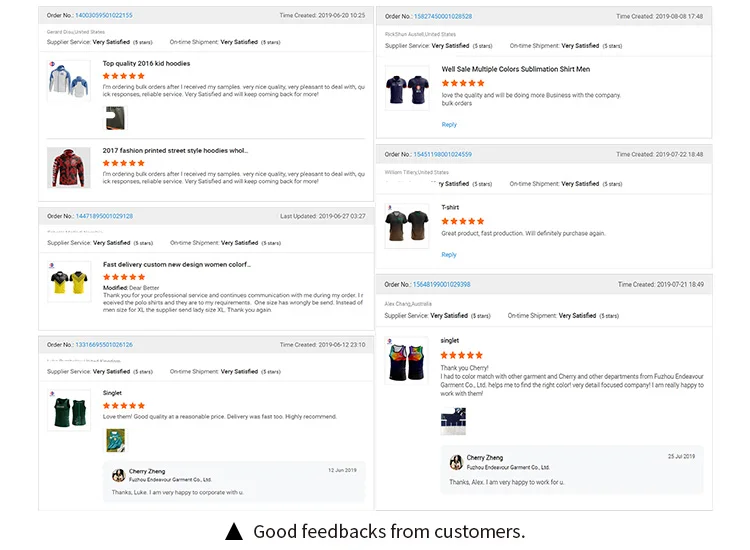A detailed view of a webpage displaying customer feedback and order details. The first order section features a grey header labeled "Order Number," followed by a set of categorized boxes summarizing the feedback. Each category includes ratings such as "Very Satisfied" and "5 Stars." Specific items reviewed include "2016 Kid Hoodies" with top ratings for supplier service, on-time shipment, and overall quality. Another product under this order is "2017 Printed Street Style Hoodies," also receiving 5-star ratings. Below this, there’s another order, though the number is too small to discern, updated as of 6-27-2019. This latter order includes a "Custom New Design" shirt, described as yellow with black accents, which also received commendations for fast delivery and quality.